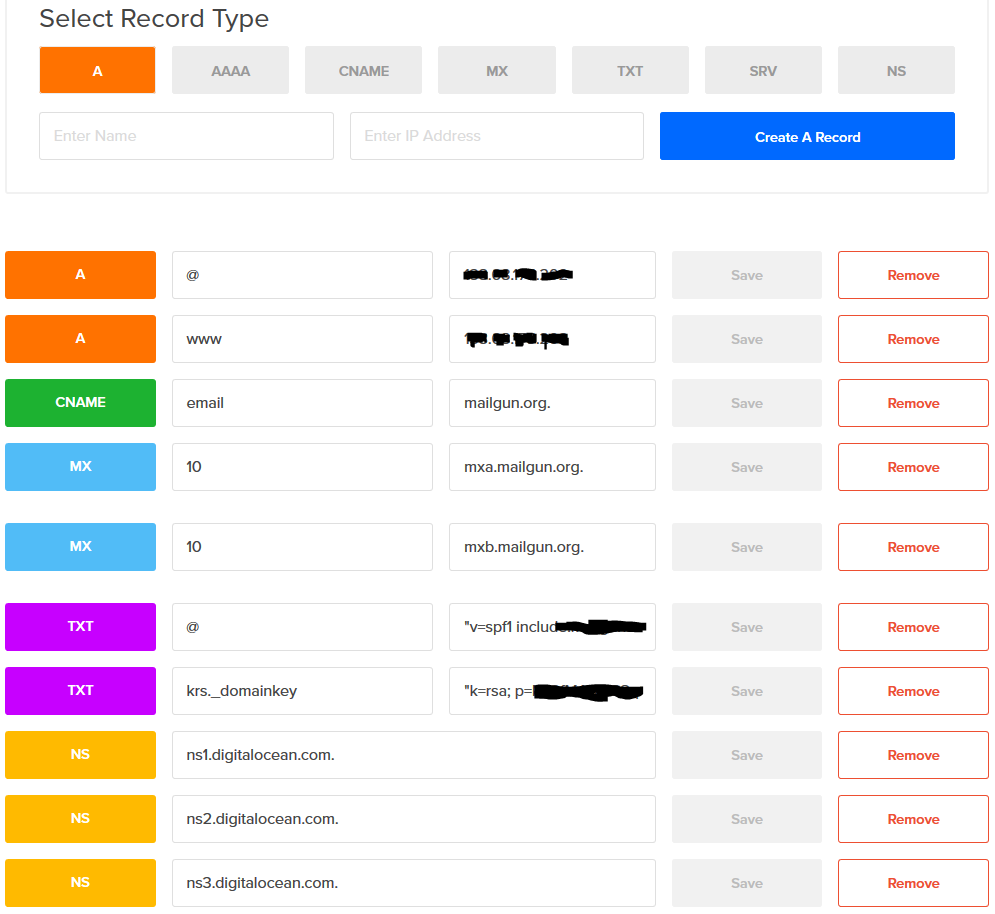The image displays a detailed user interface for managing DNS (Domain Name System) records. At the very top, there is a navigation bar with a dropdown filter labeled "Select Record Type." This dropdown includes options for various record types, arranged left to right in separate boxes. The first option, "A," is highlighted in orange, while the rest are in light gray with dark gray text: "AAAA," "CNAME," "MX," "TXT," "SRV," and "NS."

Below this filter, there are two adjacent input fields. The left one is labeled "Enter Name," and the right one, placed centrally, is labeled "Enter IP Address." To the right of these fields is a vivid blue button with white text, labeled "Create a Record."

Under these options, there is a listing of DNS records, formatted into 10 rows:

1. The first row features an orange "A" box, followed by boxes labeled "@" and a blacked-out box, then buttons labeled "Save" and "Remove."
2. The second row also has an orange "A" box, with boxes labeled "www" and another blacked-out box, followed by "Save" and "Remove" buttons.
3. The third row displays a green "CNAME" box, with boxes labeled "email" and "mailgun.org" followed by "Save" and "Remove" buttons.
4. The fourth row features a blue "MX" box, with boxes labeled "10" and "mxa.mailgun.org" followed by "Save" and "Remove" buttons.
5. The fifth row is similar, with a blue "MX" box, boxes labeled "10" and "mxb.mailgun.org," and "Save" and "Remove" buttons.
6. The sixth row has a purple "TXT" box, with a box labeled "@" and a partially obscured text starting with "(v=spf1 include)," followed by "Save" and "Remove" buttons.
7. The seventh row shows a purple "TXT" box, with a box labeled "krs.domainkey" and another box showing partially obscured text beginning with "(k=rsa; p=)," followed by "Save" and "Remove" buttons.
8. The eighth row has an orange "NS" box, with a box labeled "ns1.digitalocean.com," followed by a blank box, then "Save" and "Remove" buttons.
9. The ninth row features a yellow "NS" box, with a box labeled "ns2.digitalocean.com," followed by a blank box, then "Save" and "Remove" buttons.
10. The tenth row also shows a yellow "NS" box, with a box labeled "ns3.digitalocean.com," followed by a "Save" and "Remove" button.

Overall, the interface is designed to help users filter, search, create, and manage various DNS records in a highly organized manner.